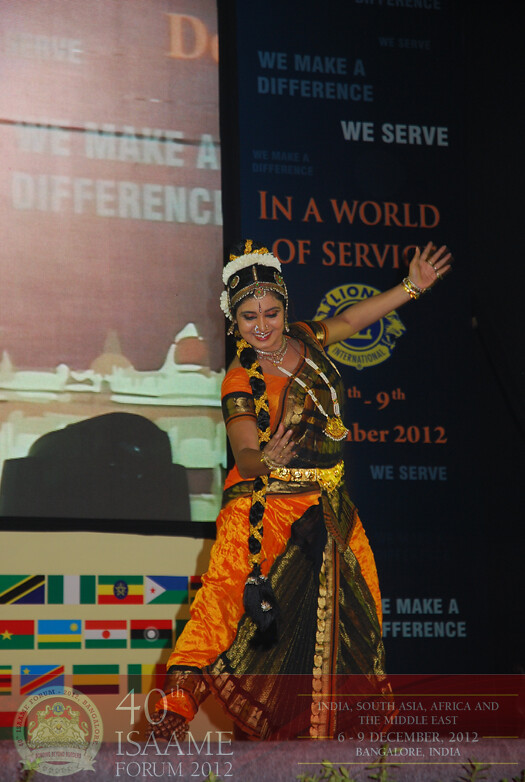The image depicts an Indian woman performing a dance on stage, captured in mid-movement with one arm gracefully extended and one leg stretched out. She is adorned in an elaborate outfit that features bright oranges, yellows, and golds, accessorized with numerous belts, scarves, and gold bracelets. Her ensemble includes a striking black and white headdress with intricate designs and a decorative braid on her left side. Prominently displayed behind her is a large, detailed backdrop with the phrases "We make a difference, we serve in a world of service," alongside multiple international flags and dates. Additionally, a semi-transparent bar at the bottom of the image reads "40th ISAAME Forum 2012," specifying the event took place from December 6th to 9th, 2012, in Bangalore, India, covering regions like India, South Asia, Africa, and the Middle East. The backdrop also features the logo of the Lions Club International.